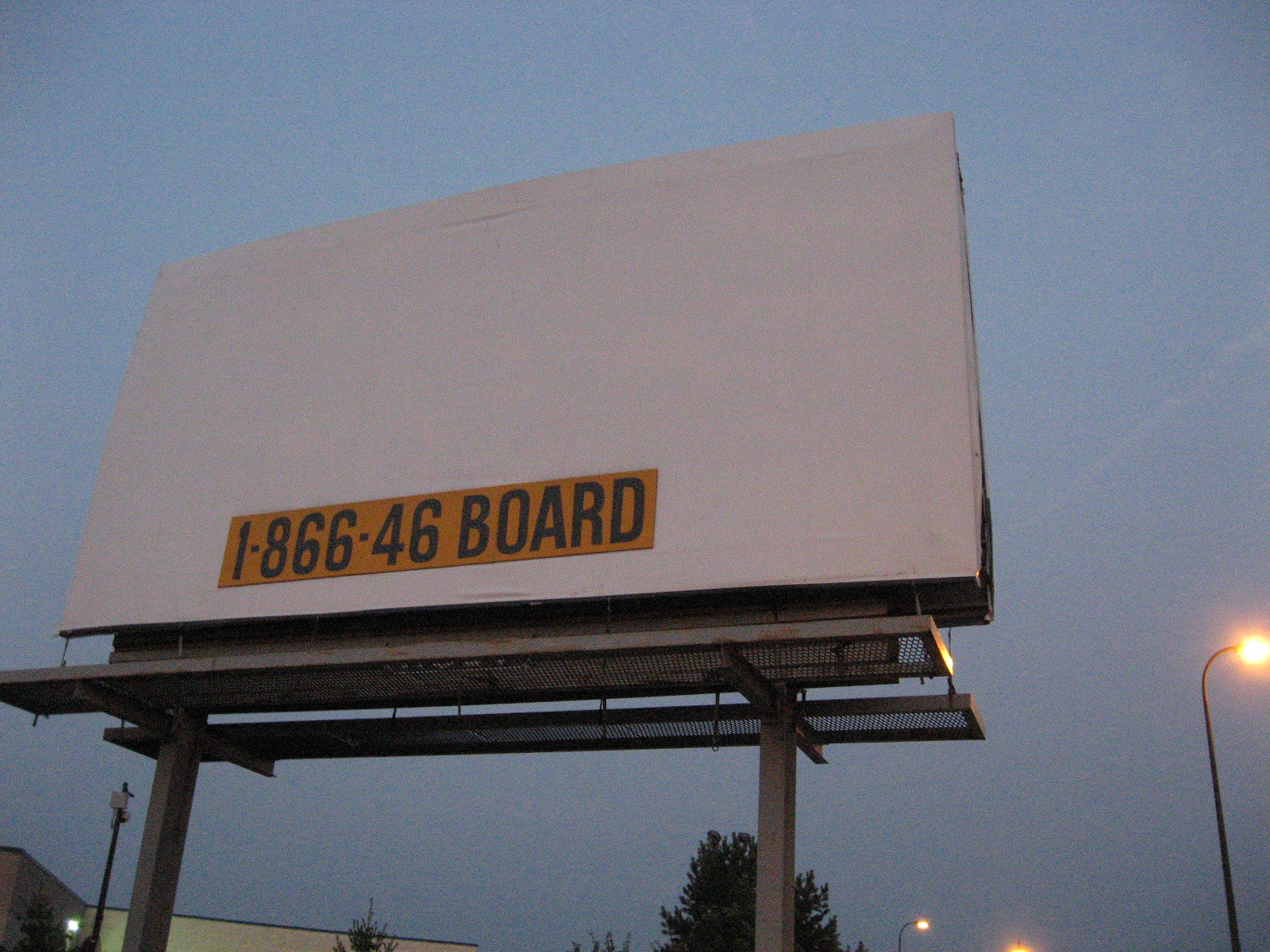In the photo, the primary focus is a large white billboard displaying the text "1-866-46-BOARD." Positioned slightly to the center-left, the billboard is situated in a setting that suggests it might be alongside a road or highway. Surrounding the billboard are various elements that add depth to the scene. 

Behind the billboard, there are three tall trees with dark green leaves, and prominently visible are four lights, possibly street or parking lot lights, giving off a yellow-orange glow. The sky in the background has a gradient of darkening blue, indicative of dusk. The top of a building can also be seen in the distance, adding an urban touch to the otherwise natural surroundings. 

Subtle details include a touch of rust on the platform of the billboard, likely where maintenance workers stand to place new advertisements. The combination of colors - blue, orange, white, black, green, and yellow-orange - paints a vivid picture of an evening scene transitioning from day to night.